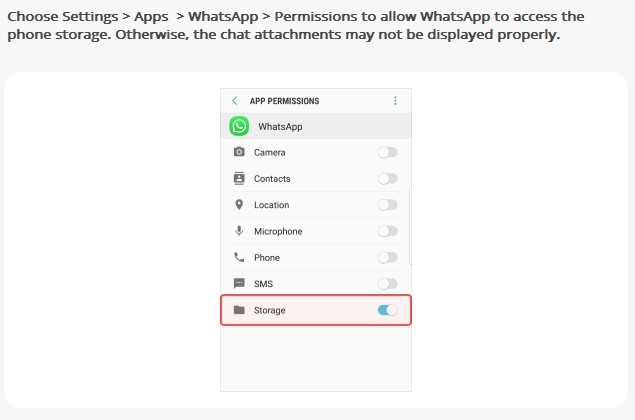The image depicts a webpage interface with details about managing app permissions on a smartphone. At the top of the webpage, there's a light gray border that is thinner on the sides and bottom. Inside this border is a line of black text which reads: "Choose settings" followed by a forward-facing arrow, then "Apps" followed by another forward-facing arrow, "WhatsApp," another forward-facing arrow, and finally a message: "Permission to allow WhatsApp to access the phone storage. Otherwise, the chat attachments may not be displayed properly."

Central to the webpage is a screenshot of a smartphone screen displaying the app permissions settings for WhatsApp. The screen's top border has a left-facing arrow, followed by the text "App permissions," and three vertical blue dots on the far right. Below, the screen lists various permissions entries in vertical order:
- WhatsApp logo followed by the text "WhatsApp."
- A camera icon next to the text "Camera," with the button in the "off" position.
- A contacts icon next to the text "Contacts," with the button in the "off" position.
- A location icon next to the text "Location," with the button in the "off" position.
- A microphone icon next to the text "Microphone," with the button in the "off" position.
- A phone icon next to the text "Phone," with the button in the "off" position.
- An SMS icon next to the text "SMS," with the button in the "off" position.
- Highlighted in red, a storage icon next to the text "Storage," with the button in the "on" position.